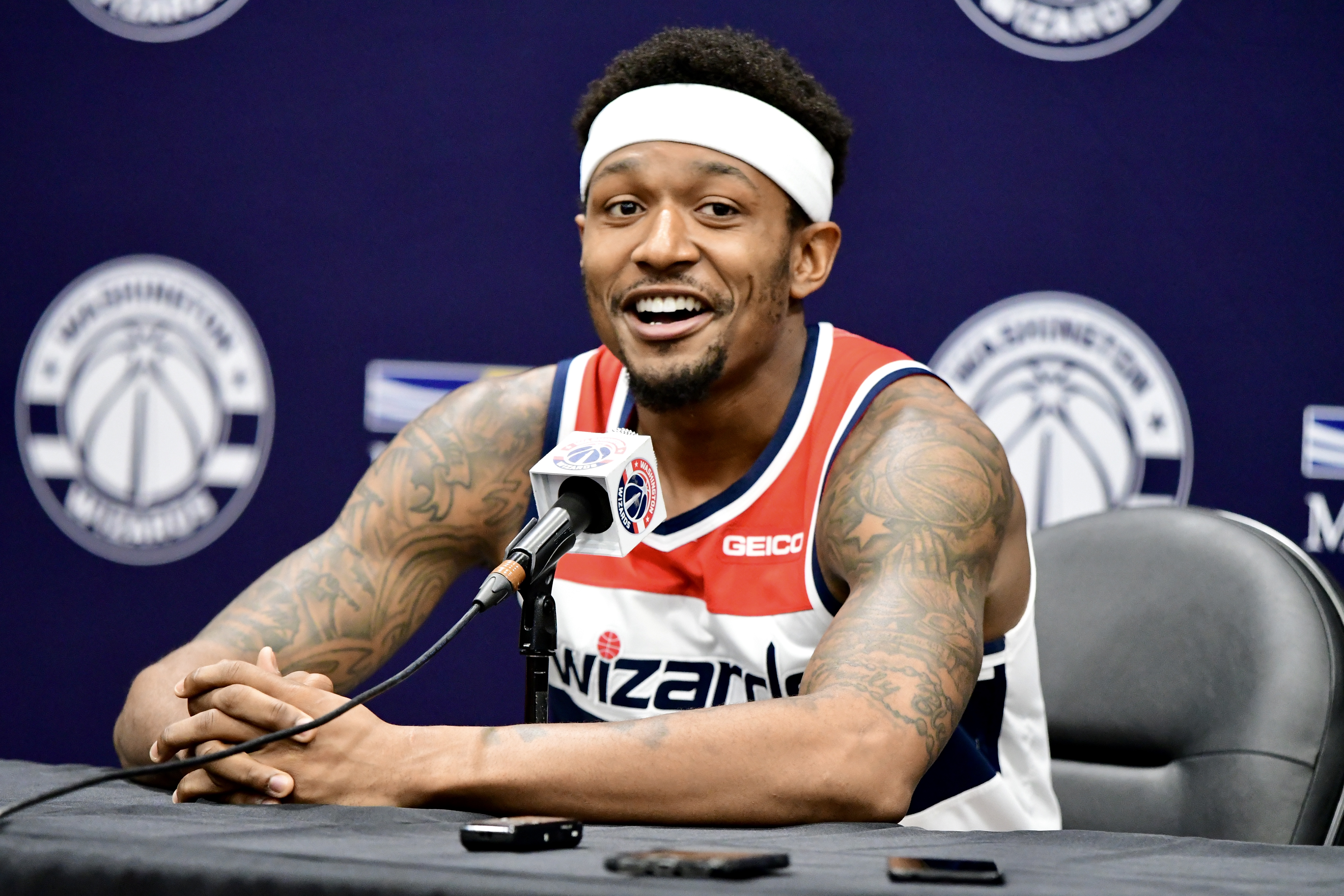In this image, a smiling black basketball player is seated at a desk, positioned centrally in what appears to be an indoor post-game conference setting. He's wearing a white and red Wizards jersey with "Geico" on the top left and a white headband. His arms are tattooed, and he has slight facial hair. The player is leaning forward with his hands on the desk, talking into a microphone that is placed close to his face. The desk is covered with a gray tablecloth, on top of which lie a couple of objects, possibly foams. Directly behind him is a gray chair. The background features a black banner with blurred-out writing and a poster that is too blurry to read. The visible colors in the image include blue, white, black, brown, gray, and red.